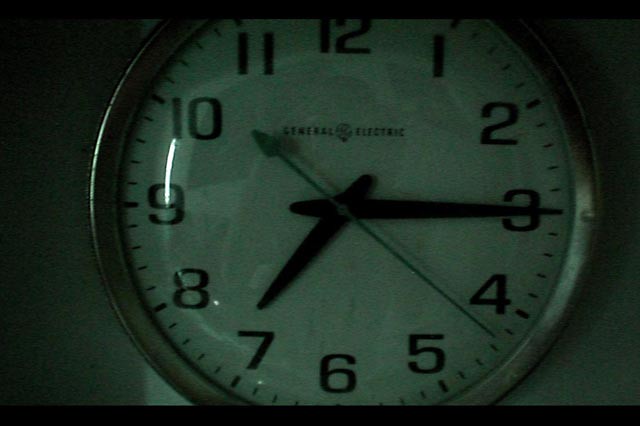The image is a close-up, slightly cropped indoor color photograph of a wall clock mounted on a white wall. The overall tone of the photograph is dark, with a faint greenish tint, and it's slightly out of focus and grainy. The clock, encased in a chrome-colored rim, reads 7:15, with the long minute hand on the 3, the short hour hand on the 7, and the second hand positioned at 22 seconds (just after the 4). The clock face features black numbers and hash marks, black hour and minute hands, and a light green second hand. Above the clock hands, the General Electric logo is clearly visible in white lettering, despite some blurriness. A reflection on the clock's plastic cover faintly reveals the silhouette of the person who took the picture. The photo has dark edges, particularly at the top and bottom.